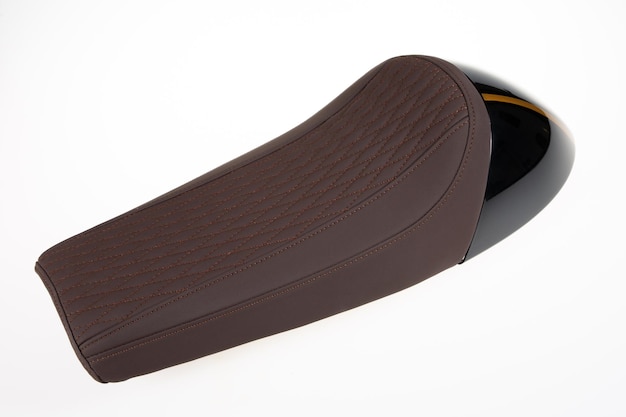The image depicts a motorcycle seat cover set against a white background, showcasing its features in detail. The seat cover is crafted from a rich chocolate brown leather, with the central portion adorned with a quilted diamond-shaped embroidery, providing both visual appeal and added texture. The leather on the sides remains plain, adding a sleek contrast to the detailed middle. The back of the seat cover features a sleek black segment accented with two parallel stripes in a light orange or yellow, adding a dash of vibrant color. The cover appears to taper slightly, suggesting ergonomic support, and the rear side exhibits a smooth, shiny plastic hull, reminiscent of the sleek finish of a helmet. Overall, the intricate pattern, rich materials, and thoughtful design elements accentuate the quality and functionality of the motorcycle seat cover.